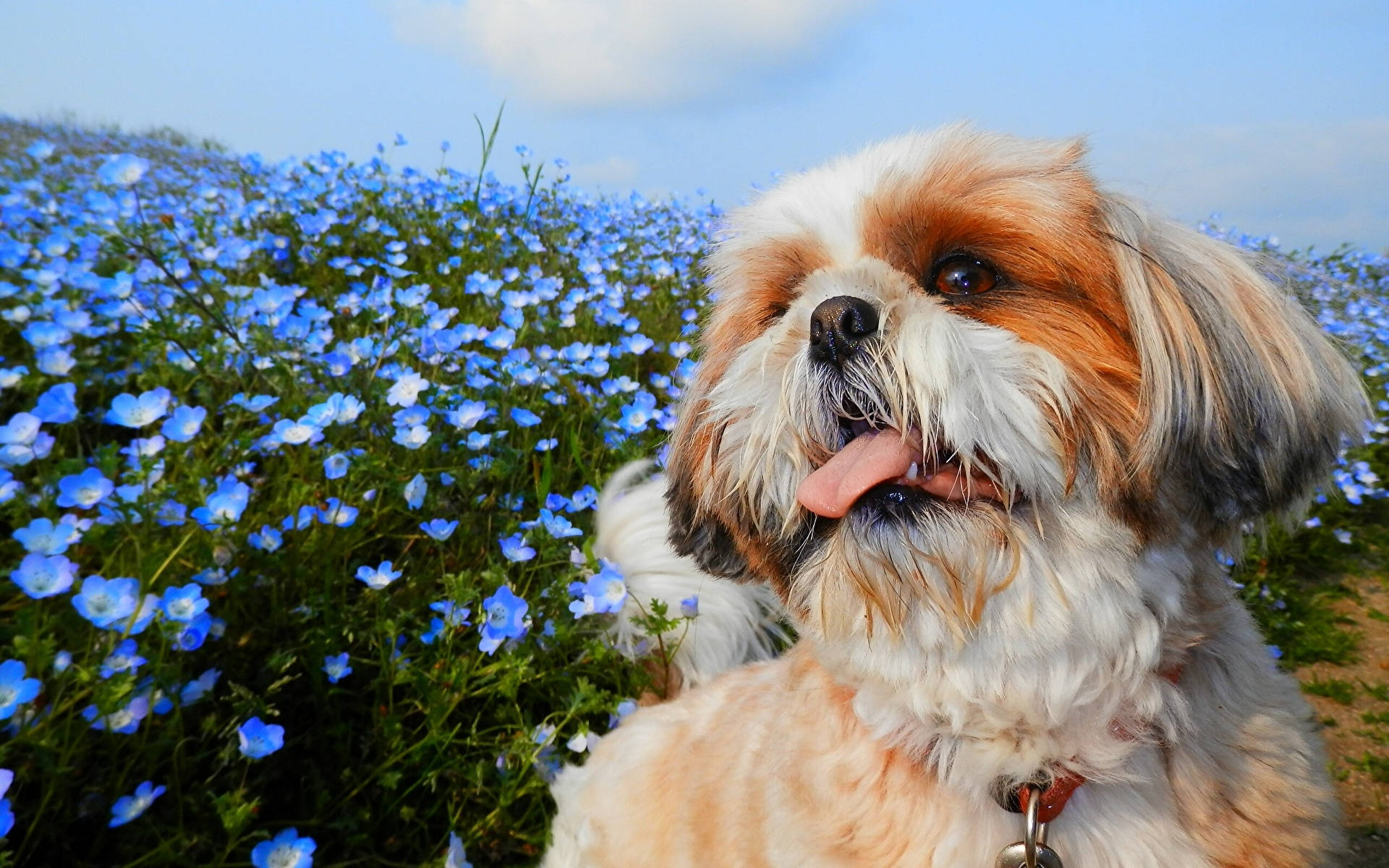The color photograph is a stunning, horizontally oriented landscape featuring a long-haired, brown and white dog in the lower right corner. This small dog, possibly a Pekingese, gazes upwards with its mouth open and tongue hanging out, revealing one of its lower teeth. It wears a red leather collar, partly hidden by its fur, with a silver tag dangling from it. The dog's brown eyes and black nose stand out clearly. In the background, a field of vibrant blue cornflowers stretches across lush green grass and leaves, filling the scene from the left bottom corner to the right side of the image. Above this picturesque floral landscape is a blue sky punctuated by a single whitish-gray cloud. Additionally, there is a small patch of dirt visible to the right of the dog.